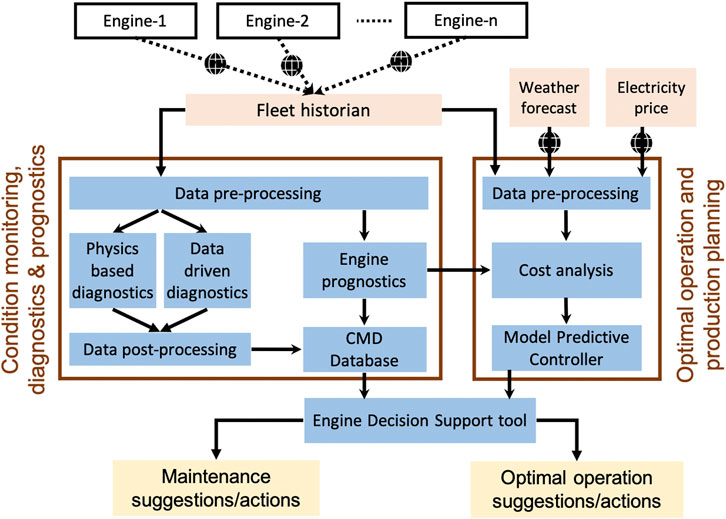The diagram is a detailed color flowchart that illustrates the process of optimizing engine fleet operations using multiple data inputs. At the top, three boxes labeled "Engine 1," "Engine 2," and "Engine N" are connected by dashed lines to a box titled "Fleet Historian." Below the Fleet Historian, two primary tracks are outlined: "Data Pre-Processing" and subsequent steps including "Physics-Based Diagnostics," "Data-Driven Diagnostics," "Data Post-Processing," and "Engine Prognostics." These processes feed into the "CMD Database" and then into an "Engine Decision Support Tool." On the left side of the chart, the terms "Condition Monitoring, Diagnostics, and Prognostics" are written vertically. On the right side, another sequence begins with "Data Pre-Processing," followed by "Cost Analysis" and "Model Predictive Controller," integrating inputs like "Weather Forecast" and "Electricity Price." This sequence aims at "Optimal Operation and Production Planning." Finally, the results of the Engine Decision Support Tool lead to either "Maintenance Suggestions/Actions" or "Optimal Operation Suggestions/Actions."